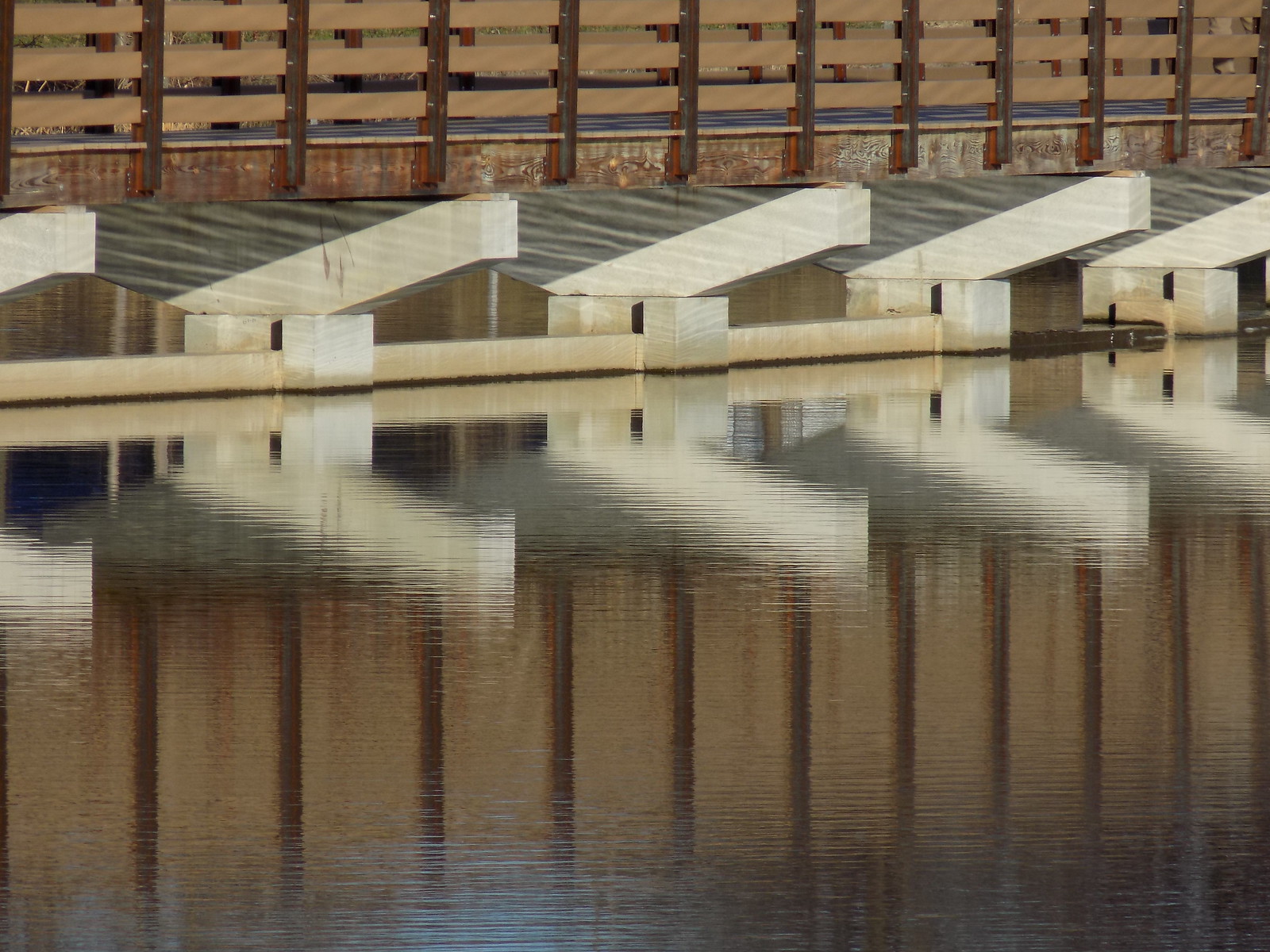The image depicts an architectural structure supporting a bridge over still, dark grey-blue water, resembling a lake rather than the ocean. Dominating the bottom 70% of the vertical rectangular shot is the calm, reflective water. Rising from the water, beginning at the 38% mark of the image, are five massive cement beams, appearing like concrete blocks stacked vertically and haphazardly toppled over. These beams support a wooden pier-like structure with weathered brown wood planks. Dark reddish-brown metal poles are vertically spaced and connected, acting as a sturdy fence to prevent people from falling into the water. Despite its aged appearance, the bridge seems in reasonably good condition, with no visible people walking along it. The overall scene exudes a serene, almost abandoned atmosphere, capturing the essence of a peaceful lakeside or riverside setting.